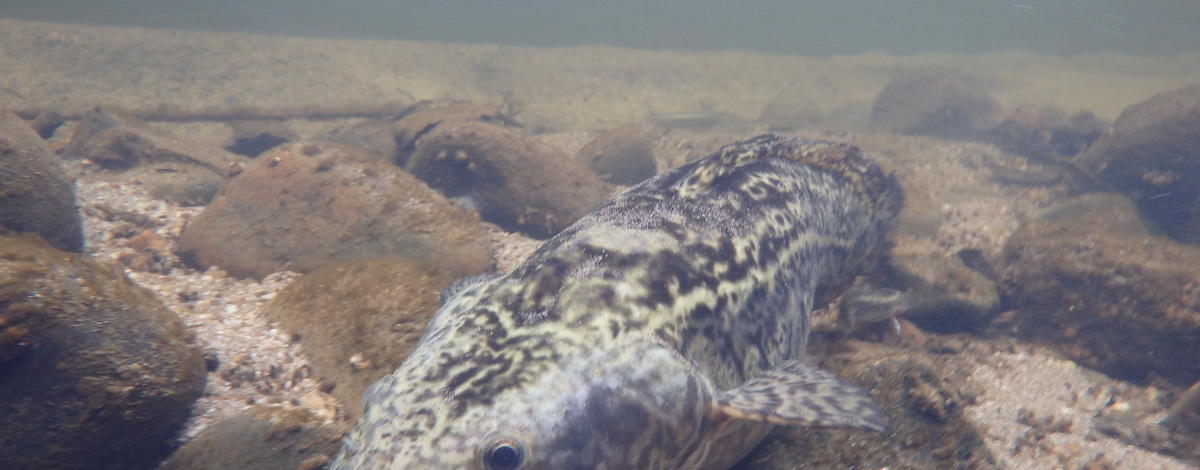In the image, a fish rests on a sandy substrate at the bottom of a body of water, surrounded by smooth brown stones with hints of green. The fish, positioned facing the southwest, is centrally located in the frame. Its body is grey with intricate black and light green patterns adorning the top, and only one of its brown and black eyes is visible. A feathery, short fin can also be seen on the right side of the image. The stones, some of which appear embedded with rounded tops, are scattered all around the fish. Fine gravel and what seems to be a cement-like structure in the background add to the underwater setting. The colors visible include various shades of gray, green, brown, and a very light peach, contributing to the overall tranquil and detailed underwater scene.